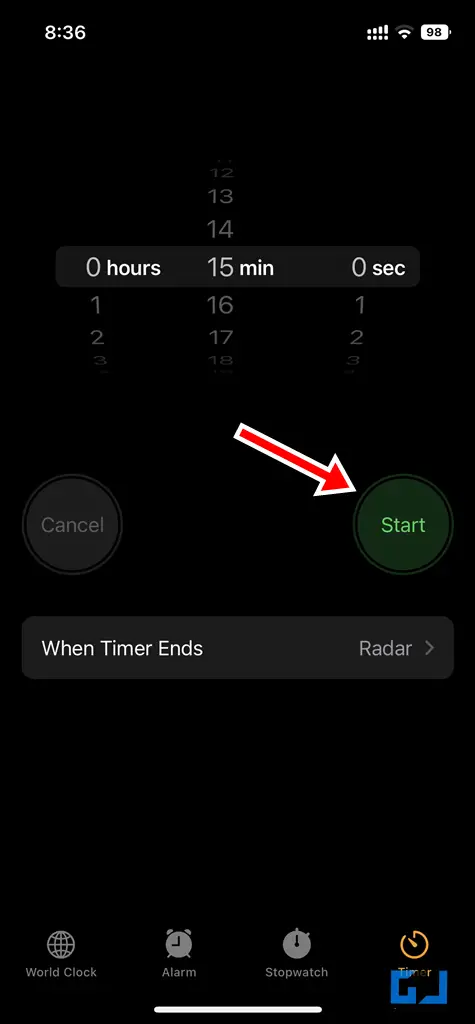This image showcases a black smartphone screen displaying a timer interface. At the top of the screen, the time is indicated as 8:36, with a battery level reading of 98%, both in white text. Below this, the timer is set to 0 hours, 15 minutes, and 0 seconds, with the hours, minutes, and seconds displayed on three separate circular wheels. On the left side of the interface, there is a large round button labeled "Cancel," while on the right, a large green button labeled "Start" is present, highlighted by a prominent red arrow pointing towards it.

Further down, a black box features white text that reads "When Timer Ends," followed by a smaller purple label "Radar," which is accompanied by a right-facing arrow. At the bottom of the screen, a black strip contains tabs labeled "World Clock," "Alarm," "Stopwatch," and "Timer." Just below, there is a logo resembling a "G" and a backwards "L" in blue, separated by a white line.